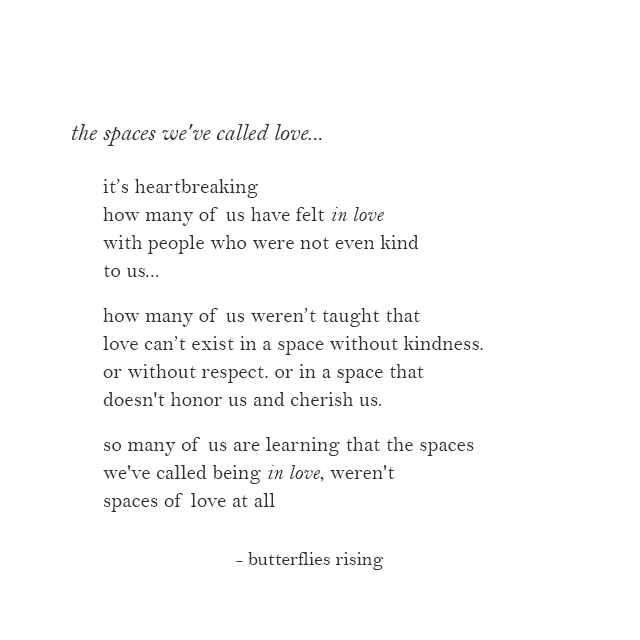Against a white background, a poem in an elegant, lowercase black font unfolds, capturing a poignant reflection on love. At the top, aligned to the left and in italics, it begins: "the spaces we've called love...". Below, slightly indented, the text continues: 

"It's heartbreaking how many of us have felt *in love* with people who were not even kind to us... How many of us weren't taught that love can't exist in a space without kindness, or without respect, or in a space that doesn't honor us and cherish us. So many of us are learning that the spaces we've called *being in love* weren't spaces of love at all."

This moving piece ends with a hyphen and the name "butterflies rising" at the bottom right, encapsulating the message of recognition and the redefinition of true love.